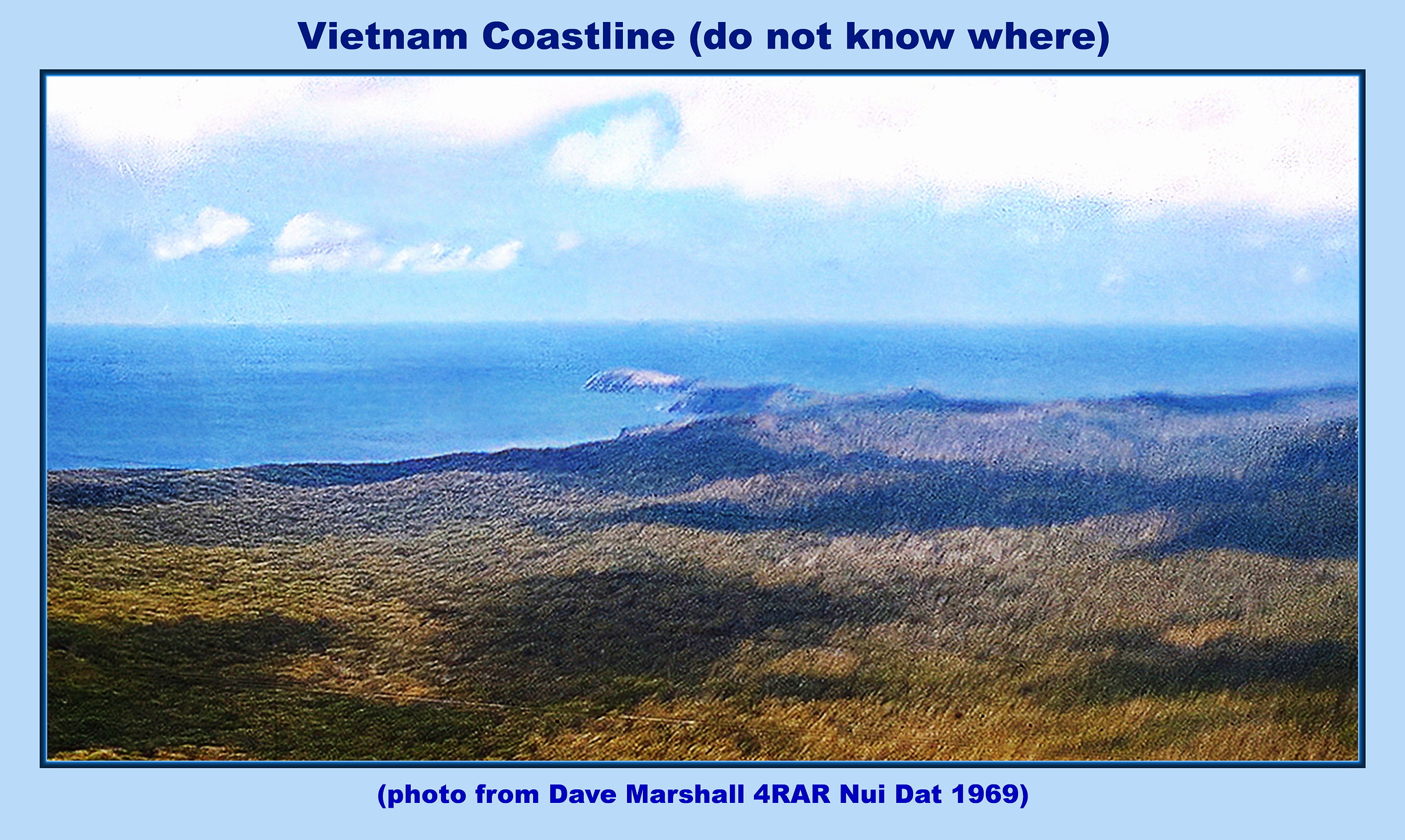In this serene, horizontally oriented photograph, the entire image is encapsulated by a thin, light baby blue border. Text in the same shade of blue adorns the border: the top reads "Vietnam coastline, do not know where," and the bottom identifies the source as "photo from Dave Marshall, 4RAR, Nui Dat, 1969." At the forefront of the landscape, a large area of lush vegetation, including grass and trees, stretches across the bottom of the photo. This verdant expanse leads to a coastline where a rocky peninsula juts out into a crystal blue ocean. Above, the sky is mostly blue, dotted with light clouds, suggesting a serene midday setting. The image showcases a harmonious palette of light blue, dark blue, white, gray, various shades of green, yellow, and tan. The entire scenic composition is centered within the frame, reinforcing its tranquil and balanced nature.